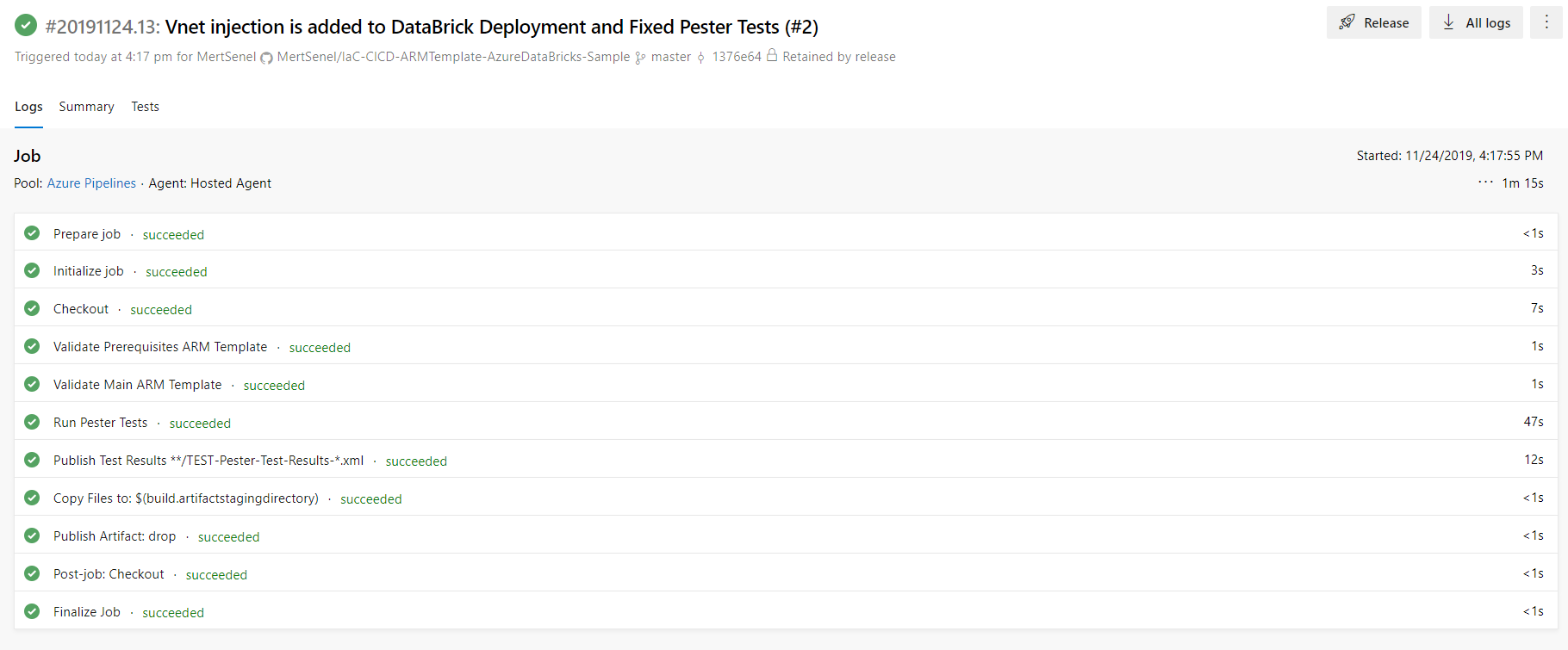A detailed screenshot description of a deployment process on a white background captures the layout and specifics of various elements and their statuses.

At the very top of the interface, there is a prominent header followed by a series of buttons. The header mentions "VNet injection is added to Databricks deployment and fixed pester test," indicating an update or action. Directly beneath the header, a timestamp reads "Triggered today at 4:17 PM."

Below the header and timestamp, there are three buttons located side by side. The first button, labeled "Release," is flanked by two other buttons: "All logs" and another button with an ellipsis, suggesting additional options.

Following this section is a detailed log summary formatted in a style reminiscent of a spreadsheet, with entries separated by subtle gray borders. The summary begins with a bold title, "Log Summary Test," and is divided into two main columns. 

Underneath the title in a gray text box, the term "Job" is displayed on the left, while the right side notes the start date as "11-24-2019" along with a specific time.

The main content consists of a list, seemingly a dozen or more items long. Each entry on the left describes a specific job or action, such as "Prepare job," accompanied by a green dot and the word "Succeeded" in green text to denote completion. On the far right of each entry is an execution time noted as “<1S,” indicating the job's duration. This pattern continues consistently down the list, providing a clear and concise overview of various tasks and their statuses.

Overall, the screenshot illustrates an organized, minimalistic interface designed for monitoring and managing deployments, with clear, color-coded indicators of task progression and status.